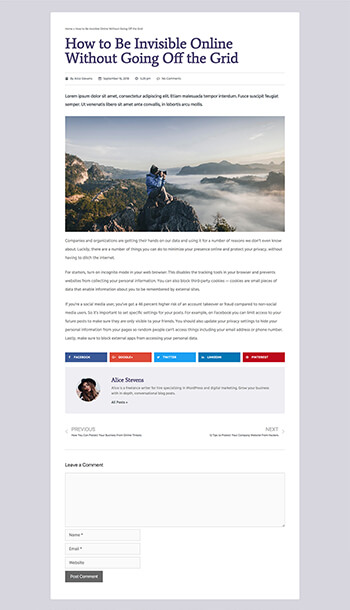The image appears to be a screenshot from a blog post titled "How to Be Invisible Online Without Going Off the Grid," with the headline prominently displayed in purple. Directly beneath the headline is a gray text box with illegible content. Following this, there are two lines of barely readable text.

The focal point of the image is a photograph featuring a person perched on a rocky mountain peak, or a similarly high and rugged surface. The individual is dressed warmly, wearing a beanie hat (often referred to as a toboggan regionally) and a blue puffer jacket. The person, also clad in gray slacks, is intently looking through the lens of a camera. Below them, a scenic view unfolds with a sea of clouds and the peaks of other mountains protruding through the misty layer in the background.

Beneath this compelling image, there are three paragraphs of text, again, not quite legible, followed by five clickable link icons at the bottom. Another gray box further down provides information about the blog's author, Alice STRVCCA, who is depicted in a small photograph as a woman with dark brown hair wearing a large black floppy hat. The details about her remain unreadable.

Below this author's blurb, navigation links labeled "Previous" and "Next" are visible on the left and right, respectively. A light gray line separates these elements from the section inviting readers to leave a comment. This section offers fields for the user's name, email, and mobile number, accompanied by a dark gray button presumed to be for submitting the comment, though its label is unclear.